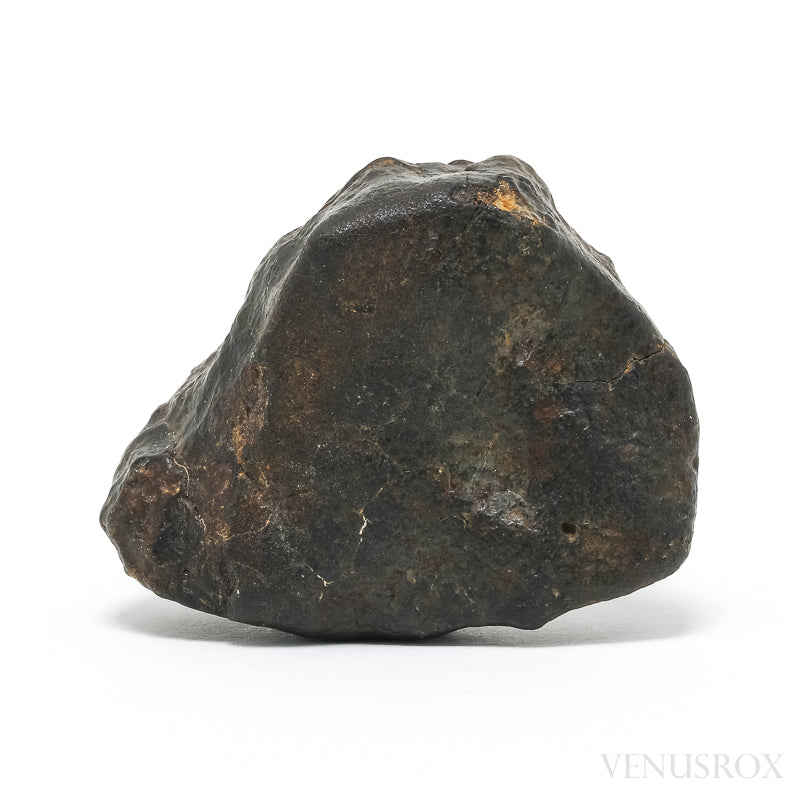The photograph showcases a large, dark rock positioned against an all-white background, accentuated by a shadow indicative of its non-flat base. A watermark at the bottom right reads "Venus Rocks" (V-E-N-U-S-R-O-X). The prominent rock is primarily dark brown to almost black, interspersed with lighter shades of gray, tan, and occasional rust-like oxidation spots. The rock displays a triangular shape with a rounded right side and a flat surface facing the camera, suggesting it has been split or cut. This exposed flat section reveals intricate textures featuring cracks, bumps, and a distinctly uneven, bumpy surface on the side turned away from the viewer. The top of the rock is particularly textural, with visible lines and irregularities, giving it an appearance almost reminiscent of a face with eyes and a nose. Despite its angular and rugged exterior, it slightly curves upward at the bottom, adding to its distinctive, layered look.